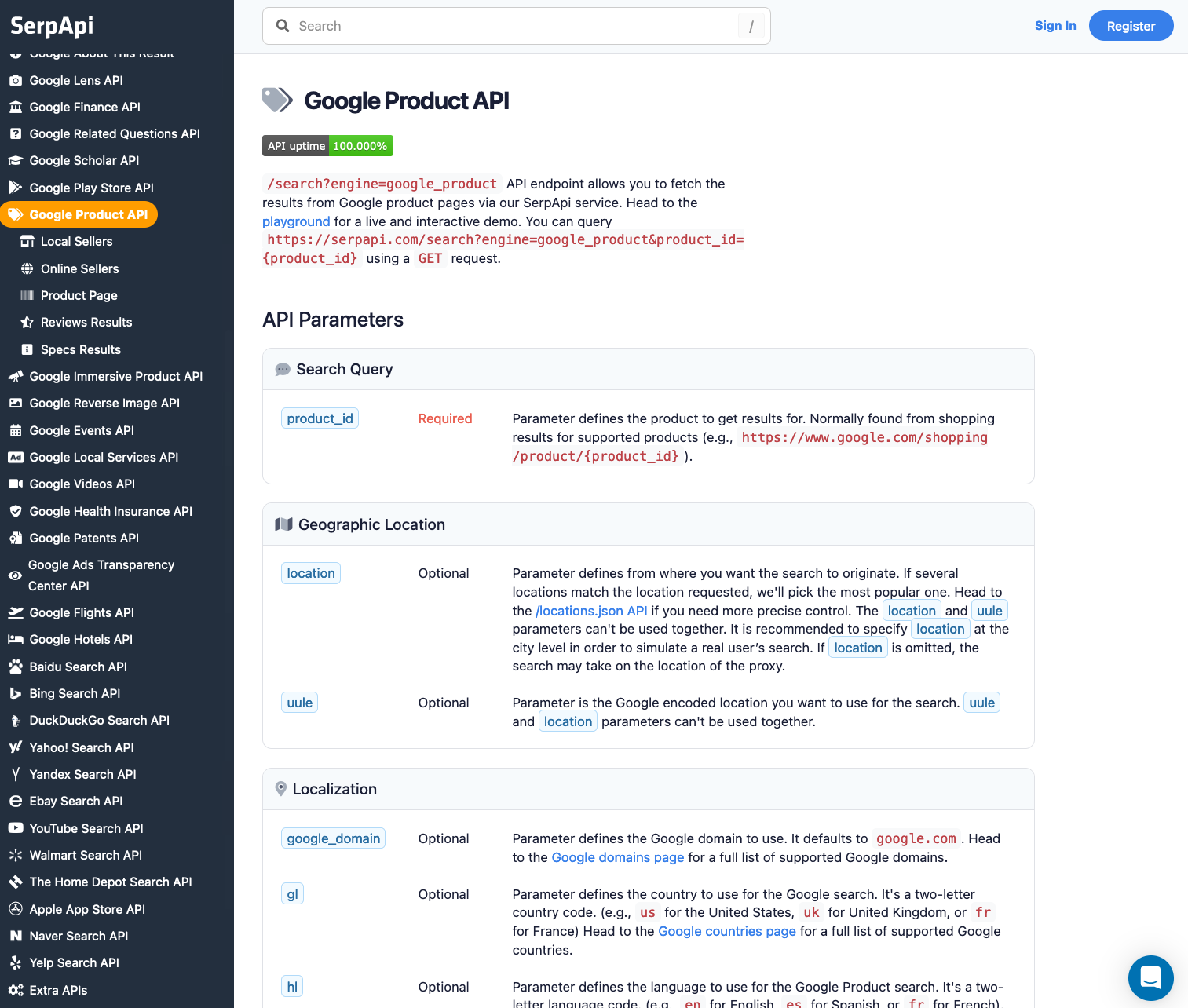This image is a detailed screen capture from a website showcasing various APIs. The screen has a dark navy background on one side with white text displaying "SERP API" along with several icons. The icons represent different categories such as a play button, Walmart logo, stars, businesses, columns, and cameras.

The visible categories include the following:
- Google Lens API
- Google Finance API
- Google Related Questions API
- Google Scholar API
- Google Play Store API
- Google Product API (highlighted in orange)
- Local Shelters
- Online Sellers
- Product Page
- Review Results
- Specs Results
- Google Immersive Product API
- Google Reverse Image API
- Google Events API
- Google Local Services API
- Google Videos API
- Google Health Information API
- Google Patents API
- Google Ads Transparency Center API
- Google Flights API
- Google Hotels API
- Beirutu Search API
- Bing Search API
- DuckDuckGo Search API
- Yahoo Search API
- Yahoo's Yandex Search API
- eBay Search API
- YouTube Search API
- Walmart Search API
- The Home Depot Search API
- Apple App Store API
- Navver Search API
- Yelp Search API
- Extra AP percentage

The central part of the screen has a white background featuring black, red, and blue text. At the top, there’s a white search bar with a blue "Sign In" link and a blue and white "Register" box. Below this, the heading "Google Product API" is prominently displayed in red font next to a gray box and a green box.

The description mentions that the API endpoint allows users to fetch results from Google product pages via the SERAPI service and directs them to a playground for a live interactive demo. 

Further down, the screen lists API parameters in black and red font:
1. Geographic Location: Defines from where you want the search to originate, picking the most popular location requested if several are available, with a suggestion to refer to the locations JSON API for precise control.
2. Localization: Allows users to specify the location.
3. Search Query: Defines the product to get results for, typically found from shopping results for supported products.

Other details include a mix of black and blue font for additional parameter specifications. Overall, this image offers a comprehensive overview of various APIs available on the website, emphasizing their uses and configurations.